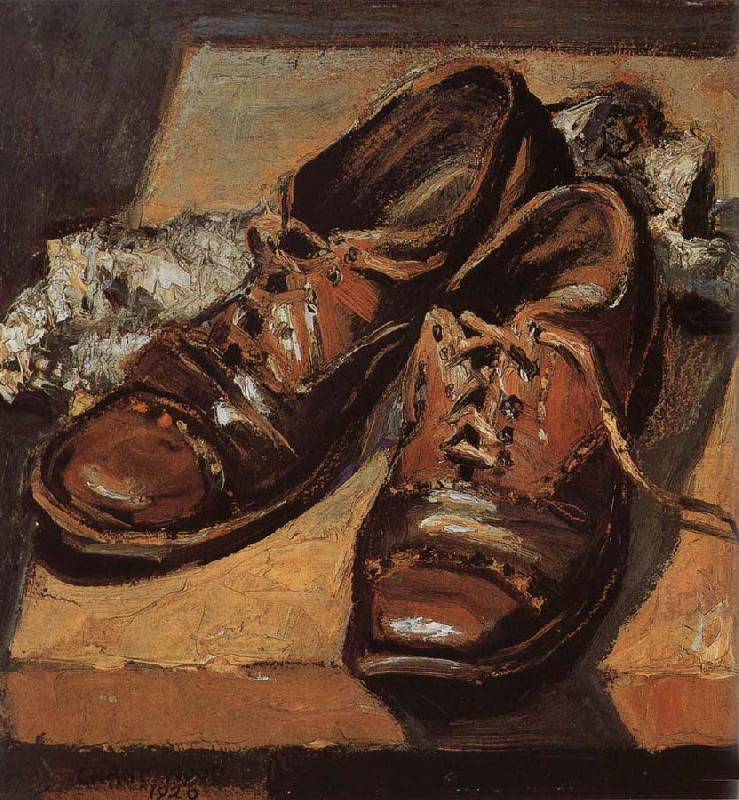This image is a detailed painting of a pair of well-worn brown leather shoes placed atop a wooden table. The shoes are characterized by their two-toned coloring, with a darker brown on the toes and a lighter reddish-brown near the areas where the laces are threaded. The leather is shiny, reflecting the light with distinct white splotches. The laces of the shoes are untied and cascading outward. The background of the painting varies with a tan whitewash on the right side, transitioning to a darker brown on the left. There is some potentially readable text in the lower left corner, possibly identifying the artist as Grant Wood and dated 1926. Beneath the left shoe's heel, there is an item that appears to be paper or socks in shades of whitish-black, grey, beige, and brown, trailing off the side of the table. The painting's edges are blacked out, further emphasizing the shoes.